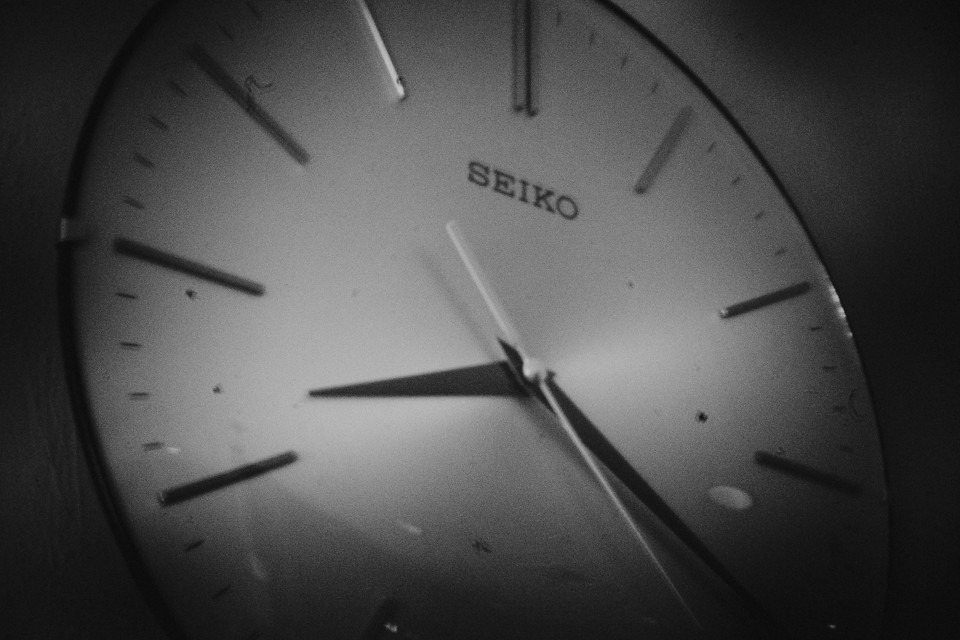A detailed black and white photograph of a Seiko clock prominently features several distinguishing elements. The clock is adorned with the company name "SEIKO" in a darker, bold font situated near the top of the lighter-colored clock face. The clock's hardware includes two dark-colored hands and one light-colored hand that point towards raised dash marks instead of traditional numbers to denote the hours. Surrounding the clock face are tiny, darker-colored dash lines that circle the perimeter, providing additional detailing. At the bottom of the clock face, there is visible dark gray shadowing along with slight dirt marks, which add an element of texture to the image. Furthermore, a subtle light reflection is noticeable on the clock face, enhancing its dimensionality.